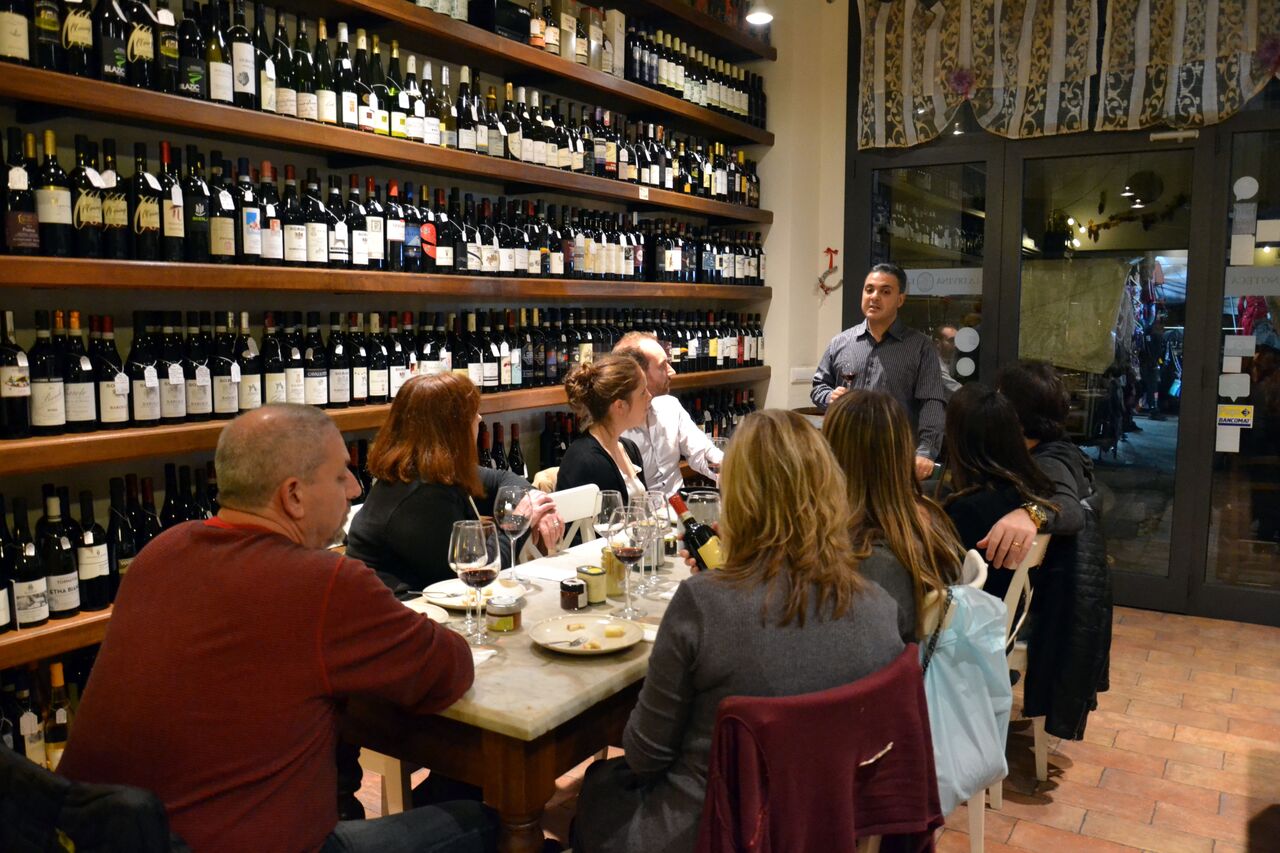In the image, a group of around eight well-dressed people is gathered in what appears to be a wine tasting venue or wine bar. They are seated at a thin table adorned with plates of food, likely cheese, and partially filled wine glasses. The entire left wall is lined with a large, fully stocked shelf of wine bottles, at least six shelves high with approximately 30 bottles each. A man with slicked-back black hair, dressed in a gray button-up shirt, stands at the head of the table next to a glass door, possibly the entrance, addressing the seated guests who all have their attention focused on him. The setting hints at nighttime, as indicated by the darkness visible through the door. The floor is light brown, possibly ceramic tile, enhancing the sophisticated atmosphere of the venue.